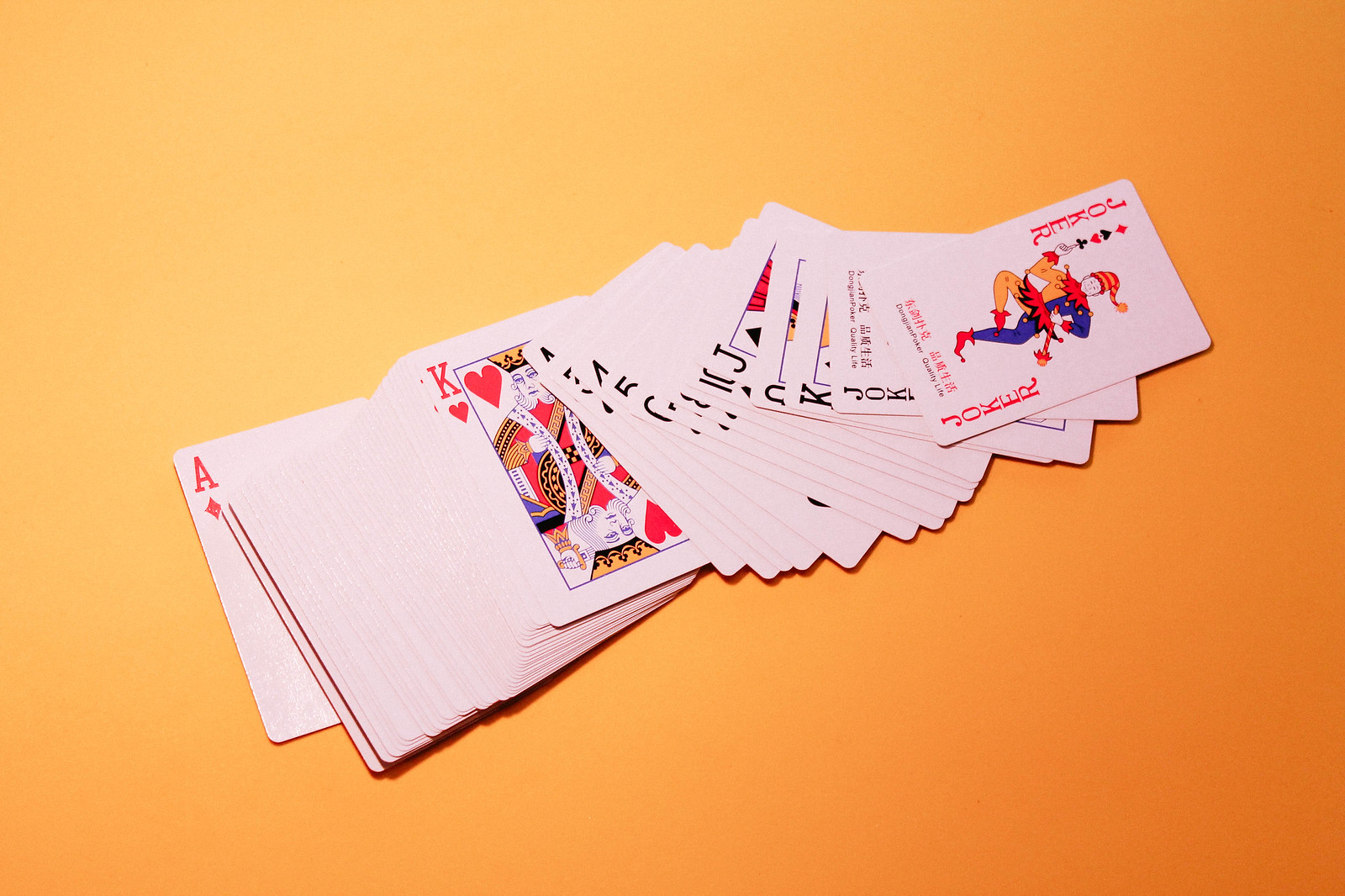The image features a spread of playing cards against an orange background. Prominent among the visible cards are the Ace of Diamonds and the King of Hearts. Additionally, there are two Jokers, each with distinct characteristics: one with red lettering and the other with black lettering. The Jokers are multicolored, with one side of their attire in orange and the other side in blue, and they wear stocking caps. Other partially visible cards include a King, Queen, Jack, and Ten from a black suit, either clubs or spades. The spread of cards appears somewhat disorganized, suggesting the presence of an additional, unseen deck.